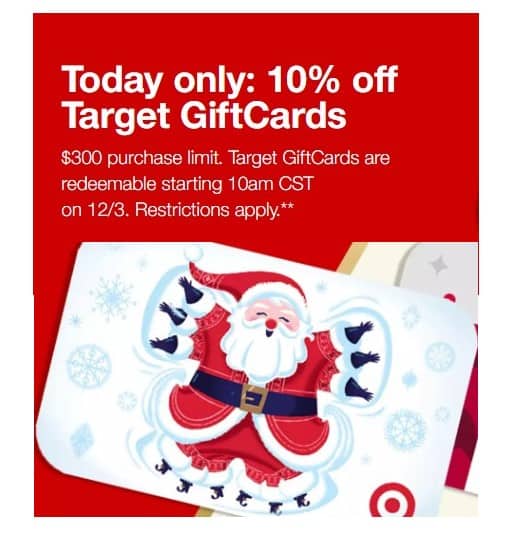This is a festive holiday advertisement from Target. In the bottom right-hand corner of the ad, in the same corner as the gift card, is the recognizable red and white Target logo. The background of the ad is predominantly red, exuding holiday cheer.

At the top of the ad, in bold white text, it reads "Today Only... 10% Off." Below this, the offer is further detailed with the text "Target Gift Cards." Further down, the details specify that there's a purchase limit of $300 per person, indicated with a symbol of the dollar sign followed by "300 persons limit."

The advertisement notes that Target gift cards are redeemable starting at 10 a.m. CST, with "CST" capitalized to emphasize the time zone. The offer is valid on December 3rd, indicated by "on 12-3" followed by the phrase "restrictions apply" accompanied by two asterisks for additional terms.

The visual centerpiece of the ad is the depicted gift card, which is primarily white, symbolizing snow. It is adorned with light blue snowflakes, adding to the wintry theme. Santa Claus is whimsically illustrated lying in the snow, creating a snow angel. He has a red nose akin to Rudolph the Red-Nosed Reindeer, and his limbs, which appear to be more numerous to emphasize movement, are dressed in black gloves and boots. Santa's joyful expression completes the festive scene.